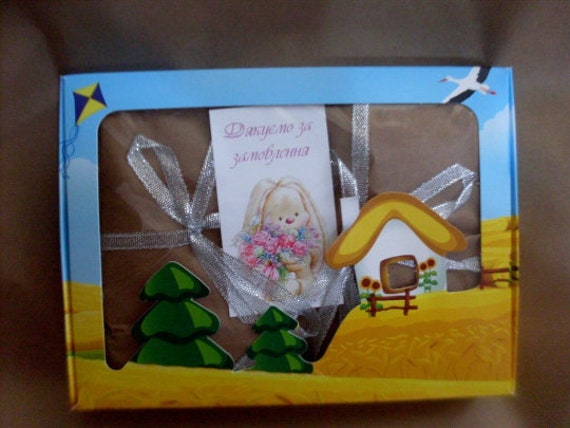The photograph showcases an intricately wrapped product, nestled within a cardboard box with a transparent plastic window on its front. The product itself is encased in a luxurious brown silky material, tied elegantly with a sheer silver ribbon. Accompanying the product, atop it, is a pamphlet adorned with a charming illustration of a stuffed rabbit with floppy ears holding a bouquet of pink, white, and blue flowers. The exterior of the box features a picturesque scene of a wheat farm, complete with a quaint white cottage with a yellow roof. The background extends into a serene blue sky, dotted with a bird with black wings soaring in the top right corner, and a yellow and blue kite fluttering in the top left. The sides of the box are further decorated with images of greenery and trees, enhancing the overall rustic and whimsical aesthetic.